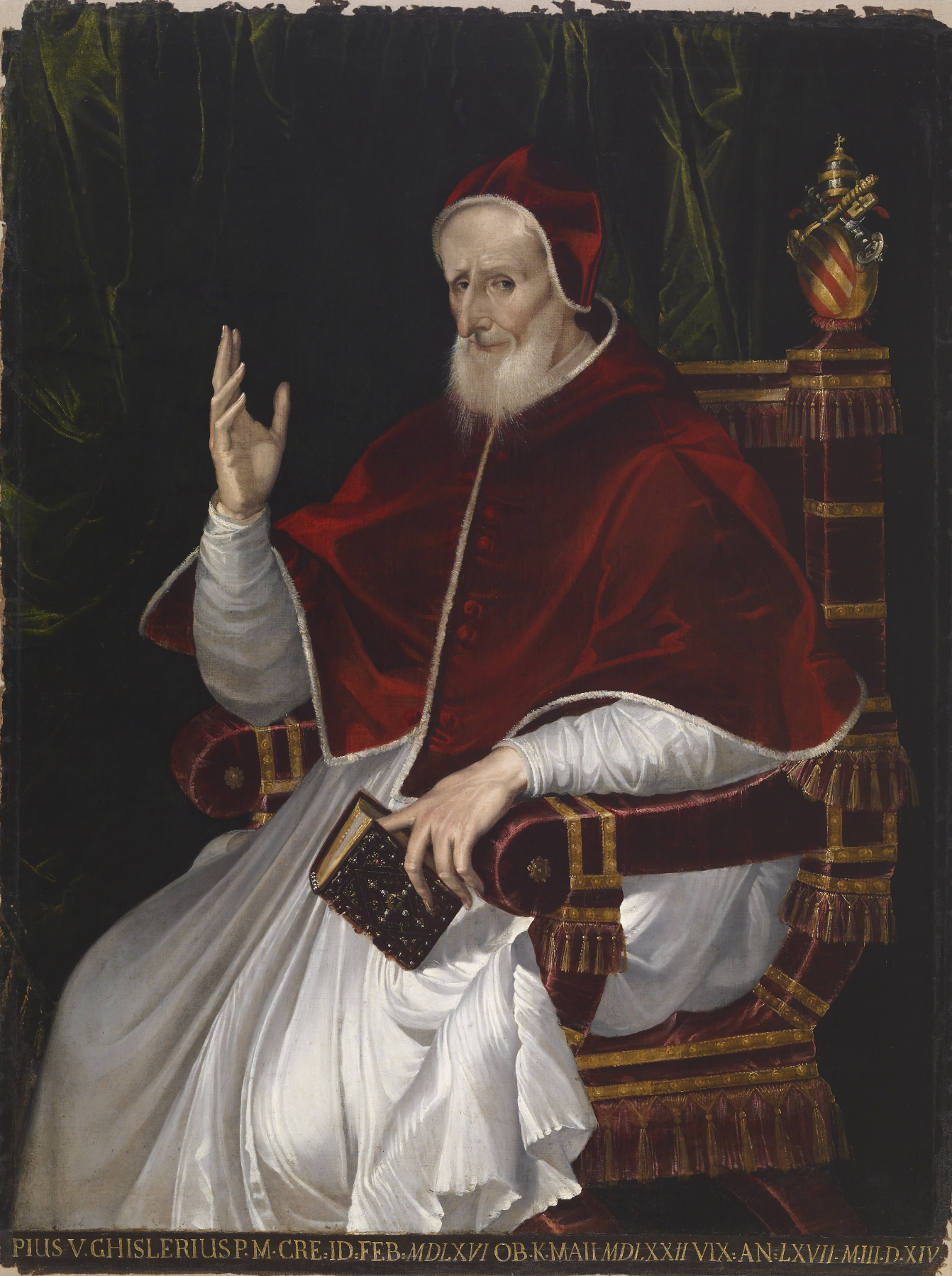The painting depicts an elderly Catholic Cardinal, likely from the Renaissance era, seated in an ornate wooden chair adorned with red velvet upholstery and gold detailing, including tassels and ornamental pin nails. The Cardinal is characterized by his gray beard and kind, yet gaunt, facial features, including a long, crooked nose. He wears a traditional white linen robe beneath a vibrant, dark red velvet tunic that lacks sleeves, and a matching red velvet hat. His left hand rests with fingers splayed on the armrest, while his right hand holds an ornate book, probably a Bible, which rests on his left thigh. The setting includes a green velvet backdrop, giving the painting an air of opulence and reverence. The chair features a crest on its upper right corner, and at the bottom of the painting, Latin text, including the name "Pius V" and Roman numerals, adds to the historical and religious context of the artwork.